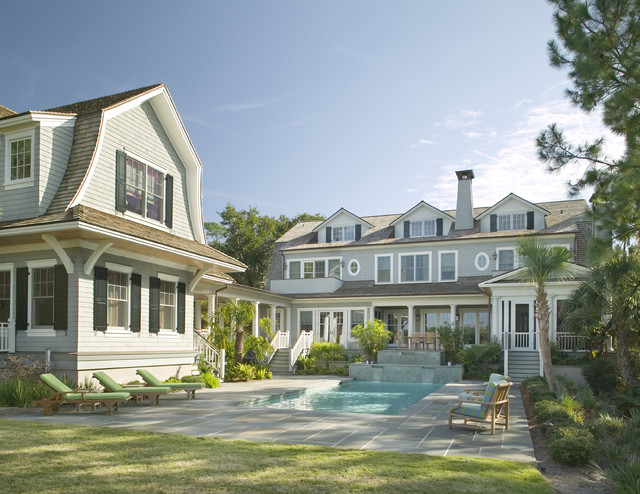This outdoor photograph showcases a luxurious backyard scene dominated by a central clear pool adorned with a couple of small waterfalls cascading over stone steps. The pool is flanked by lounge chairs: green ones on the left and blue-cushioned ones on the right. The vibrant, well-maintained green lawn in the foreground transitions into a stone walkway leading to the pool area. Behind the pool stands a tall three-story house painted in a bluish-white or grayish color, complemented by numerous windows and a set of steps leading to its first floor. To the left, there's a connecting extension with an off-white facade, appearing as either a two-story guest house or a pool house. This secondary structure is situated near a series of beach chairs. Further to the right of the main house, a line of towering trees, possibly palm trees, stretches up to the top of the image. The sky above is a serene light blue, completing the picturesque and inviting atmosphere of this plush residence.